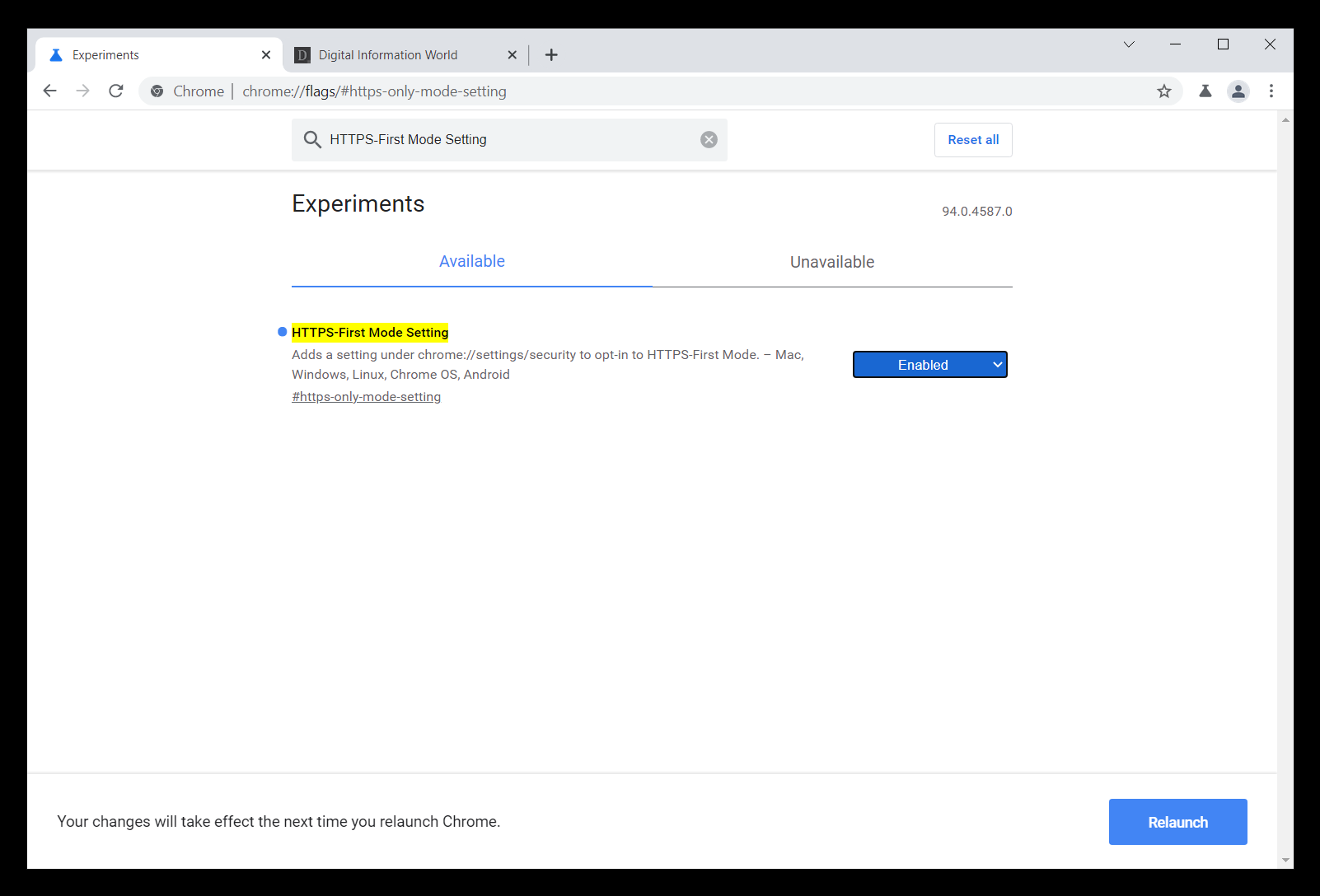Screenshot of a Chrome web page displaying the "Experiments" settings. The browser tab in the upper left shows "Experiments," and another tab, "Digital Information World," is open beside it. The active URL presented in the address bar is "chrome://flags/#https-only-mode-setting." Below the URL bar, a search field and a blue "Reset All" button are visible.

The main content area, set against a white background, features a prominent black heading labeled "Experiments." There are two menu options below this heading— "Available" and "Unavailable"—with the "Available" option highlighted in blue.

Within the "Available" section, the "HTTPS-only-mode-setting" option is prominently highlighted in yellow, marked by a blue bullet point to its left. An adjacent blue box labeled "Enabled" indicates the setting's status. In the lower right corner of the page, a blue "Relaunch" button is also visible.